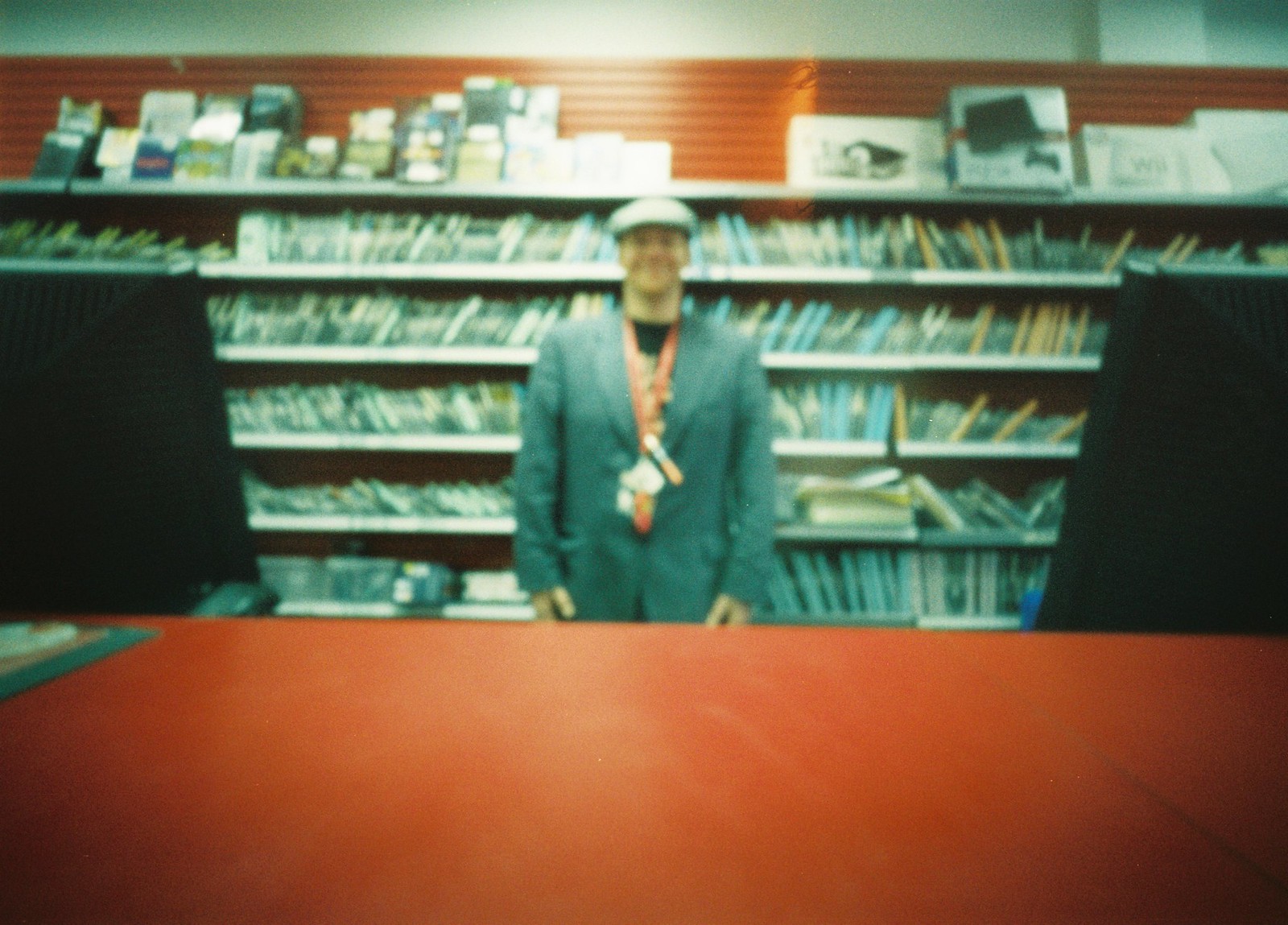In this vintage-style, blurry photograph, we glimpse the interior of a library from the perspective of a patron approaching the checkout desk. The desk stretches from the lower left to the right corner of the image, crafted from a brown material that adds to the antiquated atmosphere. At the center of the frame stands a librarian, donned in a gray suit jacket over a black t-shirt, with a bright red lanyard around his neck and a small cap atop his head. Although his fair-skinned features are indiscernible due to the blurriness, his professional attire is evident. Behind him, six white bookshelves are crammed with books of various colors, including blues, yellows, reds, whites, and blacks, some leaning slightly left or right, giving a sense of a well-used and loved collection.